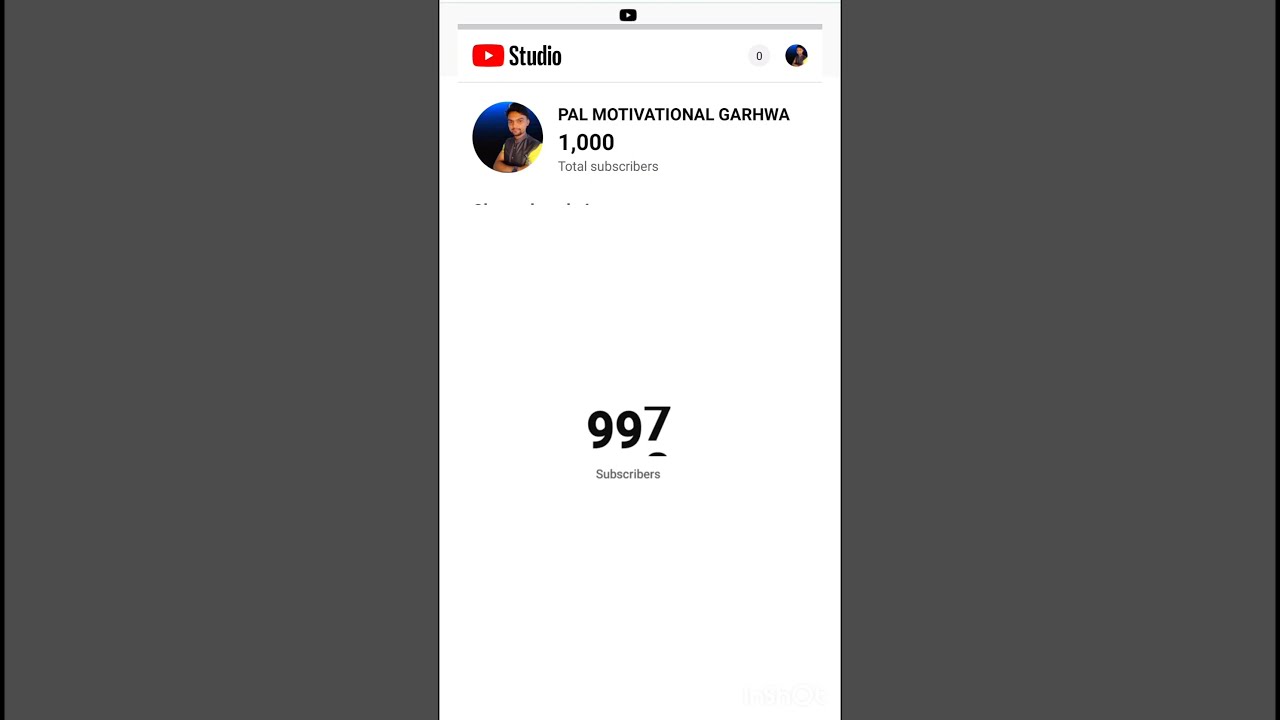The image is a detailed screenshot of a YouTube channel page. On the top left, it features the iconic red play button logo of YouTube, next to the word "Studio" in black text. On the top right corner, there is a circular icon showing the channel user's profile picture – a man with black hair, a black beard, and mustache, with his arms crossed, possibly of Middle Eastern descent. Just below this, the channel name "Pal Motivational Garhwa" is displayed, accompanied by "1000 total subscribers." Dominating the center of this vertical rectangular screenshot is a dynamic subscriber counter, currently fluctuating from 997 towards 998. This main screenshot section is bordered by a solid gray background, highlighting it like a prominent vertical strip amidst the entire green backdrop of the image.